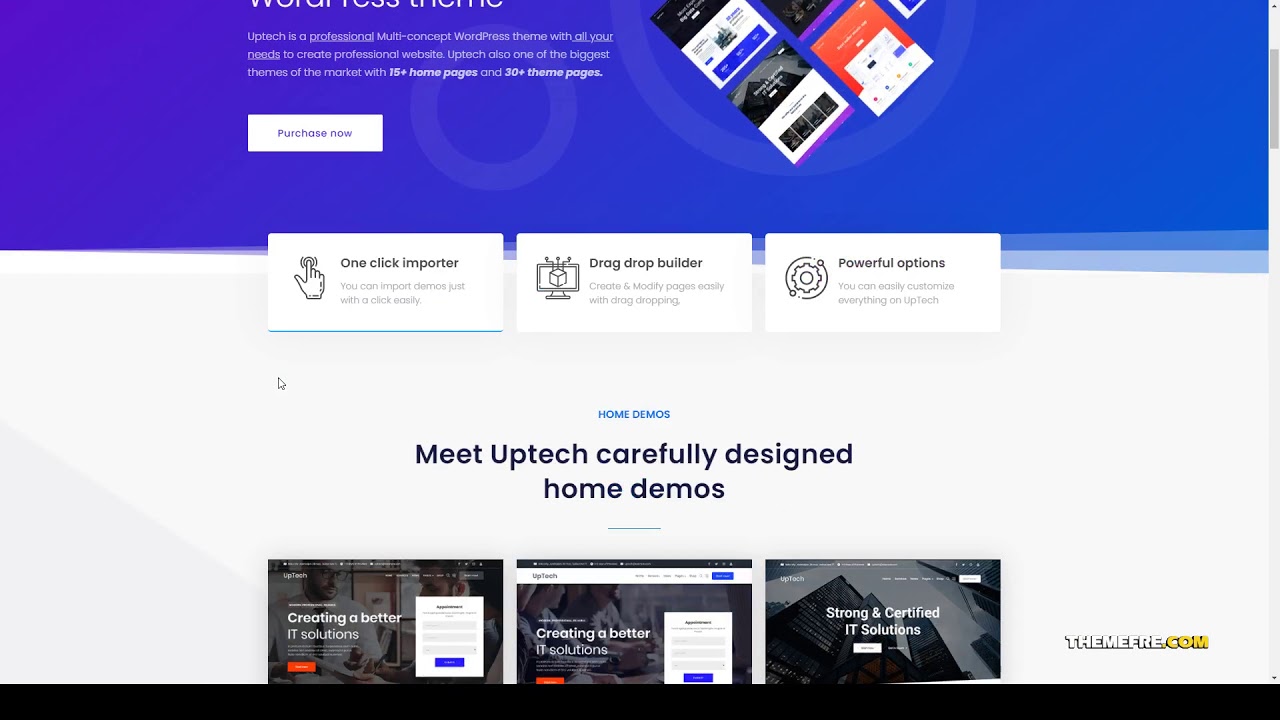This is a detailed screenshot of a promotional webpage for the Murphree Company, emphasizing the features of the Uptek WordPress theme. At the top of the page, a partially visible blue box contains text that reads, "Uptek is a professional multi-concept WordPress theme with all your needs to create professional websites. Uptek also is one of the biggest themes on the market with 15-plus homepages and 30-plus theme pages." The text is slightly cut off towards the end.

Beneath this, a prominent white box includes a compelling call-to-action: "Purchase now." As you scroll down, there are additional white boxes highlighting key features of the theme. The first box reads "One-click importer," the second states "Drag & Drop Builder," and the third indicates "Powerful Options."

Further down, in small blue letters under these feature boxes, the text "Meet Uptek, carefully designed home demos" introduces a series of sections, each with a black background and images of people engaging in various activities. The first section showcases "Creating Better IT Solutions," accompanied by an orange "Buy It Now" button. The second section repeats the same phrase and button. The third section deviates slightly with the background depicting a complex array of machines, titled "Strong and Certified IT Solutions."

At the bottom of the screenshot, there is a website address, "themurphree.com," followed by a black strip lining the bottom edge of the page.